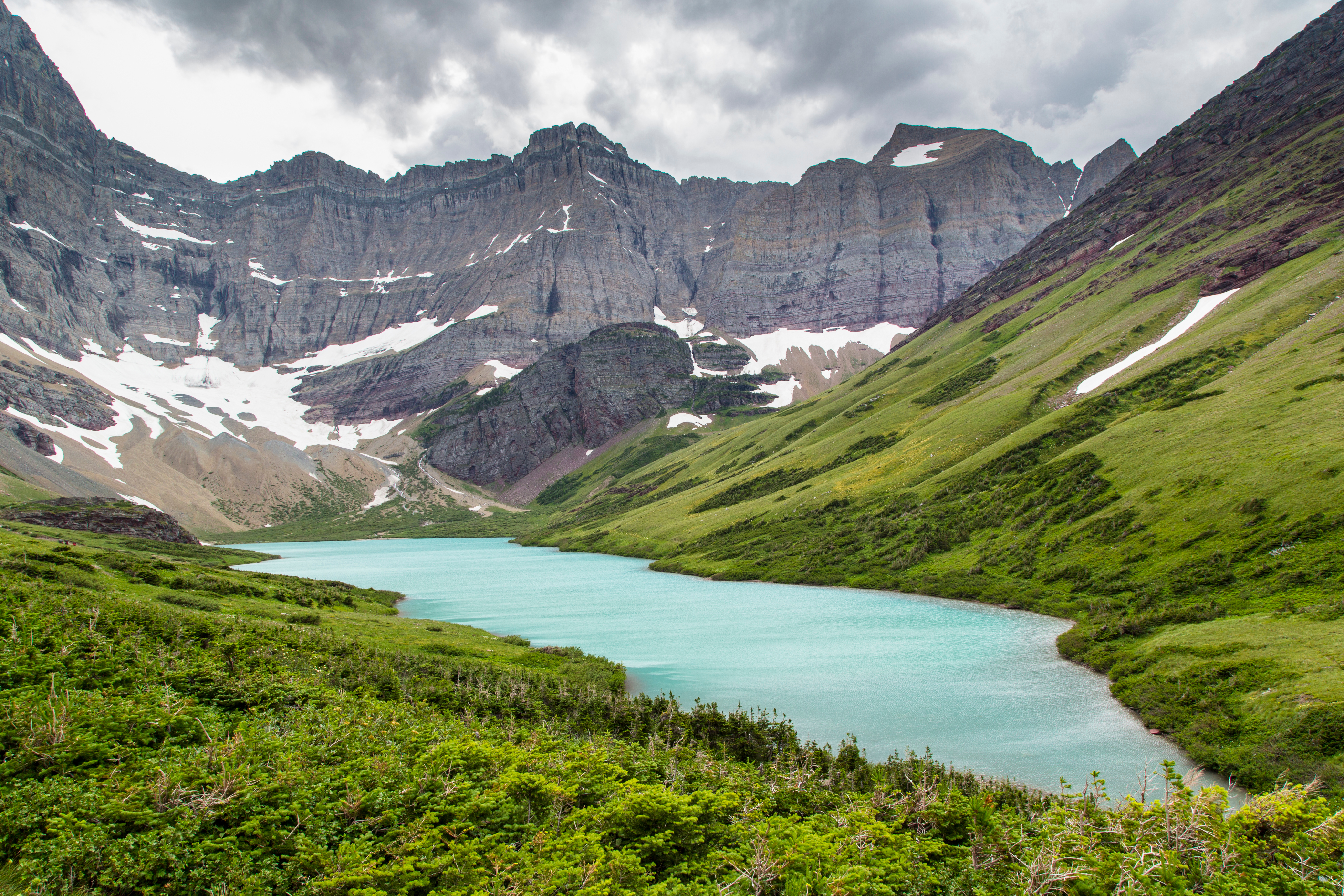The image is a full-color, square photograph capturing a serene outdoor scene during the daytime, illuminated by natural light. Dominating the upper section of the image is a cloud-filled sky, with dark gray clouds suggesting an impending rainstorm. Below the sky, a large, rugged mountain range with dark gray, weathered rocks stretches across the horizon. The mountain peaks are sprinkled with patches of snow, indicating a high elevation. 

In the foreground and to the right side of the image, a vibrant green hill covered in lush grass rises gently, with a small white patch that could be either snow or fine sand. Nestled at the lower part of the scene, towards the center, is a tranquil, teal-blue lake. This still body of water creates a striking contrast against the natural stone tones of the mountain behind it.

The lower right to the lower left section of the photograph is a grassy expanse adorned with patches of different shades of green, interspersed with vague, colorful wildflowers, adding a delicate touch to the rugged landscape. The overall composition blends the stark contrasts between rock, water, and foliage, creating a harmonious and detailed depiction of nature's beauty.